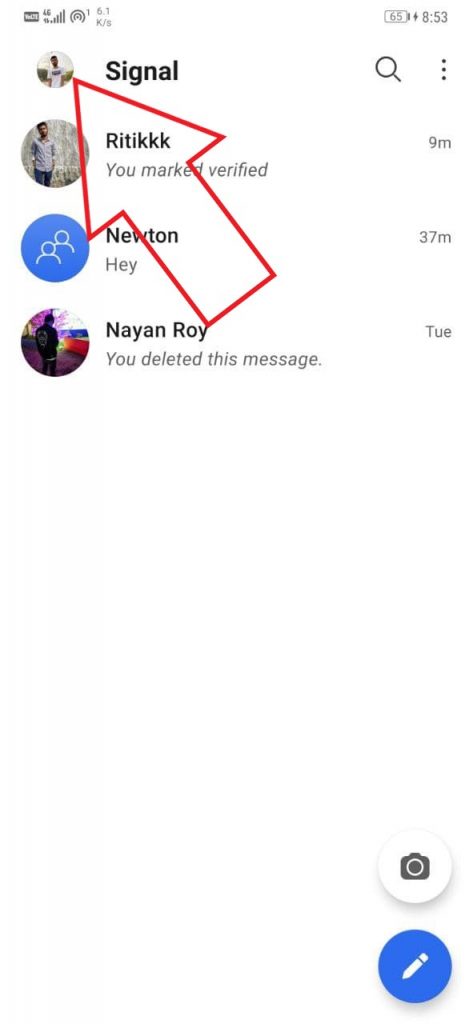The image is a screenshot from a mobile device showcasing multiple user profiles vertically stacked against a white background. At the top, there is a prominent user profile labeled "SIGNAL" in bold black text. This profile features a circular profile picture of a man wearing a white t-shirt. A striking red arrow outlines and points to this profile, drawing attention to it. 

Below the "SIGNAL" profile, there are additional user profiles. The second profile belongs to a user named "RITIKKK," depicted with a profile picture of a person in a grey shirt and blue pants. This profile is marked with a "UMACT verified" badge beneath the username.

The third profile in the sequence is simply labeled "Newton," and the final profile listed at the bottom is named "Neon Roy." Each profile is displayed in a clean, straightforward manner, maintaining the same format and contributing to a cohesive layout.